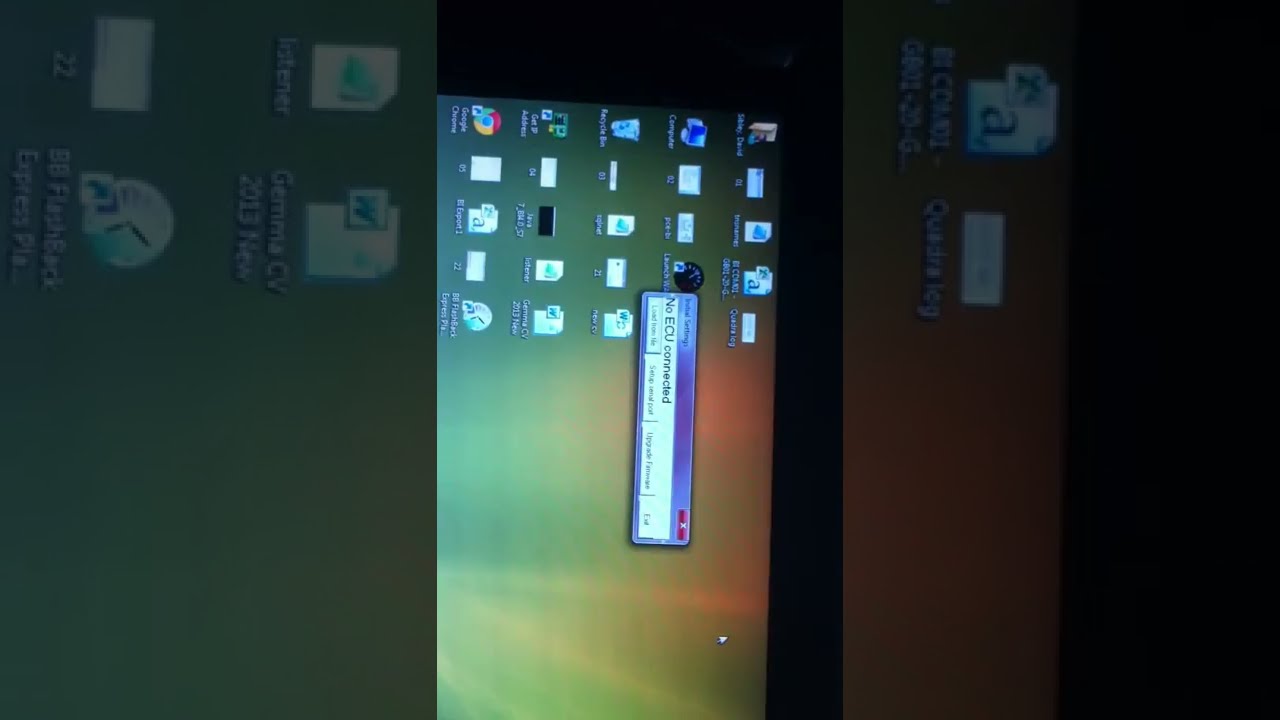The image shows a rotated screenshot of a computer monitor, tilted 90 degrees to the right. Dominating the upper left portion of the screen are various desktop icons typical of a Windows operating system, including icons for "Computer," "Recycle Bin," "Google Chrome," and several individual files. The background features muted, blended colors, transitioning from green and yellow to a spectrum that includes blue, orange, and red. Centrally, there's a small, horizontally oriented window with an informational message that reads "No ECU connected" beneath an unreadable title. A red 'X' is visible in the upper right corner of this window, indicating an option to close it. The screenshot captures a blend of close-up and distant views, with the icons becoming blurrier towards the edges.